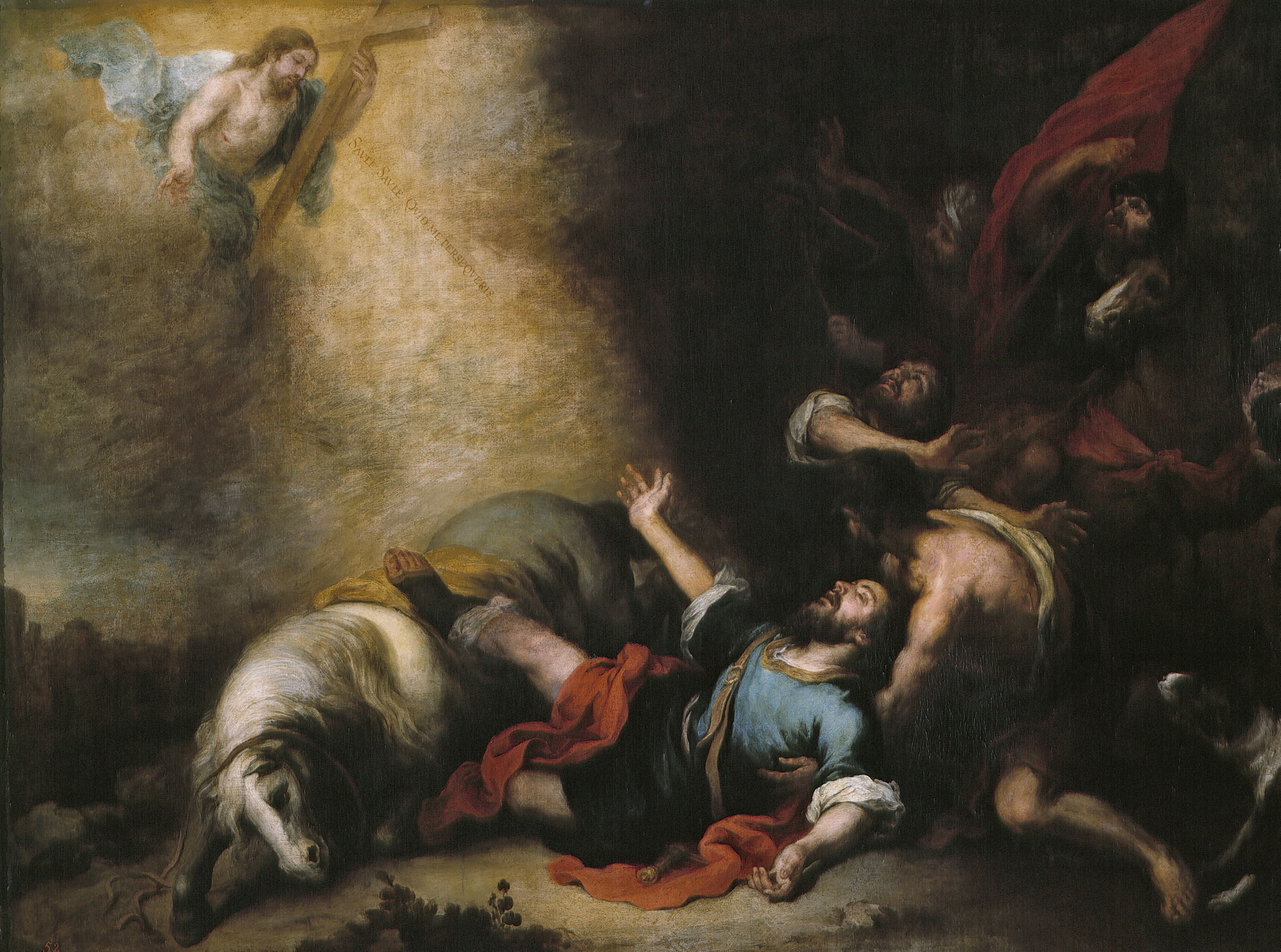The painting depicts a poignant religious scene with Jesus Christ carrying a large crucifix in the top left corner. He is depicted with traditional long hair and a beard, adorned with angelic wings, and partially draped in a flowing white robe that leaves his torso exposed. He is illuminated by a golden light that contrasts sharply with the otherwise dark brown backdrop, creating a divine aura around him. 

On the ground below, several figures are depicted in prayerful poses. Four men, adorned in regal blue, black, and red robes with intricate details, gaze upwards towards Jesus, their expressions a mix of reverence and awe. One man, appearing like a shepherd, is lying on the ground, partially supported by another figure behind him, with his leg trapped under a gray horse with a distinctive white mane and muzzle. The horse appears to be in distress, adding to the somber atmosphere of the scene.

The meticulous use of light and shadow in the painting highlights the divine presence of Jesus, bathing the central figures in a warm, golden light while casting the surrounding areas into darkness. This contrast underscores the spiritual significance of the moment, drawing the viewer's attention to the celestial vision above.